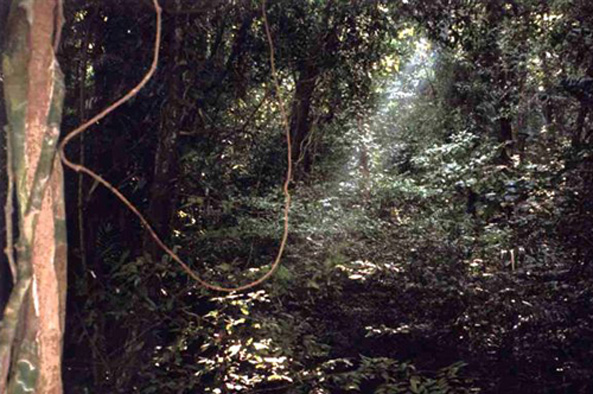The photograph captures a dense, forested area. Dominating the left side of the frame is a tree trunk with a reddish hue, wrapped in dark-colored vines, including one distinctly looped vine hanging down. The background and remaining space are filled with various shades of green from the grass, leaves, and foliage that obscure most of the branches. Sunlight pierces through the canopy, creating a focused ray of light that illuminates the forest floor. The scene is a mix of vivid greens and earthy browns from some dried leaves, presenting a lush yet slightly shadowy forest environment.